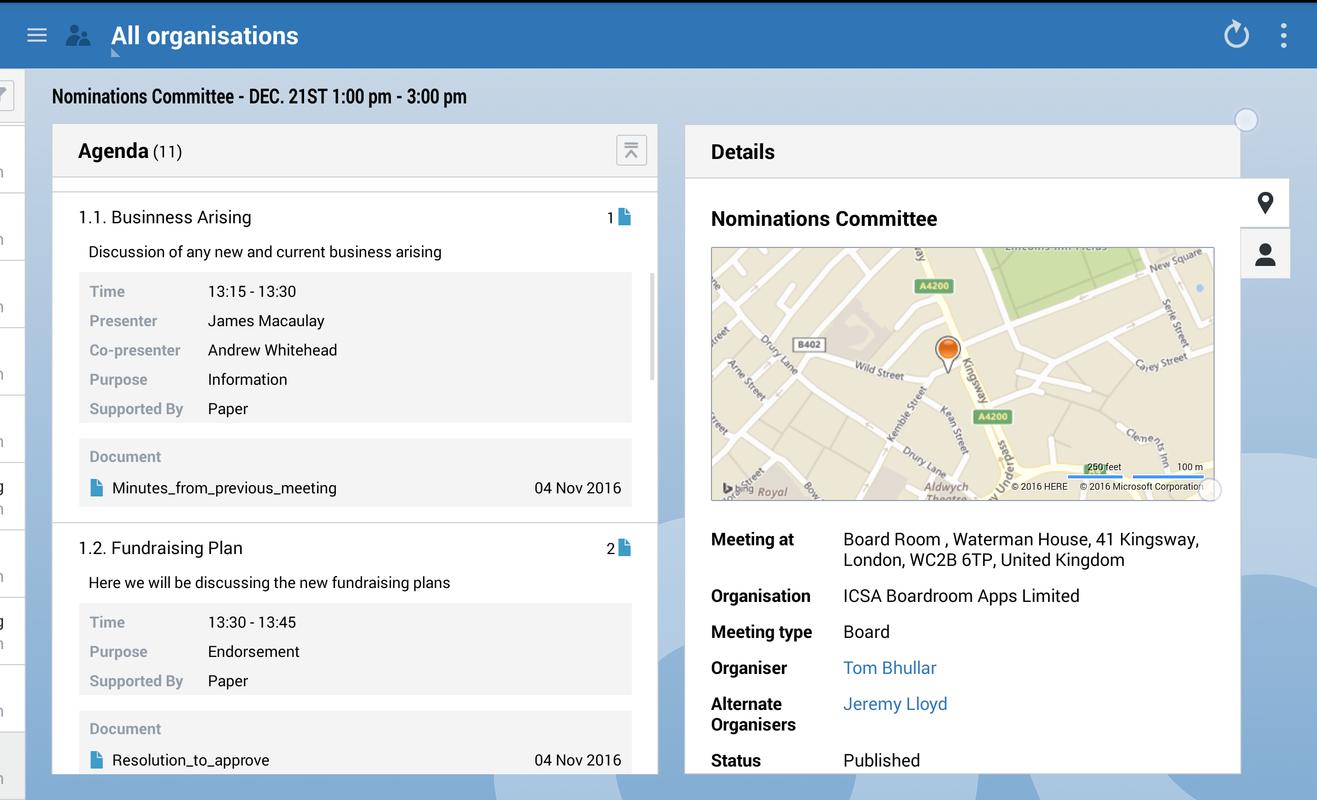The image appears to be a screenshot of an application or website interface detailing a meeting agenda for the Nominations Committee. At the top, there is a medium blue bar labeled "All Organizations." Directly below, a light blue border contains text stating "Nominations Committee December 21st 1 p.m. to 3 p.m."

Occupying most of the image are two white boxes filled with smaller gray sections. The left box is an agenda with the header "Agenda 11," listing items:

1. **1.1 Business Arising**: Discussion on any new or current business arising. 
   - **Time**: 13:15 to 13:30 
   - **Presenter**: James McCauley
   - **Co-presenter**: Andrew Whitehead 
   - **Purpose**: Information supported by paper 
   - **Document**: minutes_from_previous_meeting_04_November_2016

2. **1.2 Fundraising Plan**: Discussing new fundraising plans.
   - **Time**: 13:30 to 13:45
   - **Purpose**: Endorsement supported by paper 
   - **Document**: Resolution_to_approve_04_November_2016

The box on the right is labeled "Details" for the Nominations Committee meeting. It includes an image of a city map with an orange icon marking the location. Below, it provides the meeting specifics:

- **Venue**: Boardroom, Waterman House, 41 Kingsway, WC2B 622, United Kingdom.
- **Organization**: ICSA Boardroom Apps Limited
- **Meeting Type**: Board
- **Organizer**: Tom Bowler
- **Alternate Organizer**: Jeremy Lloyd
- **Status**: Published

This detailed caption overviews an organized yet detailed description of the meeting schedule and logistical information.